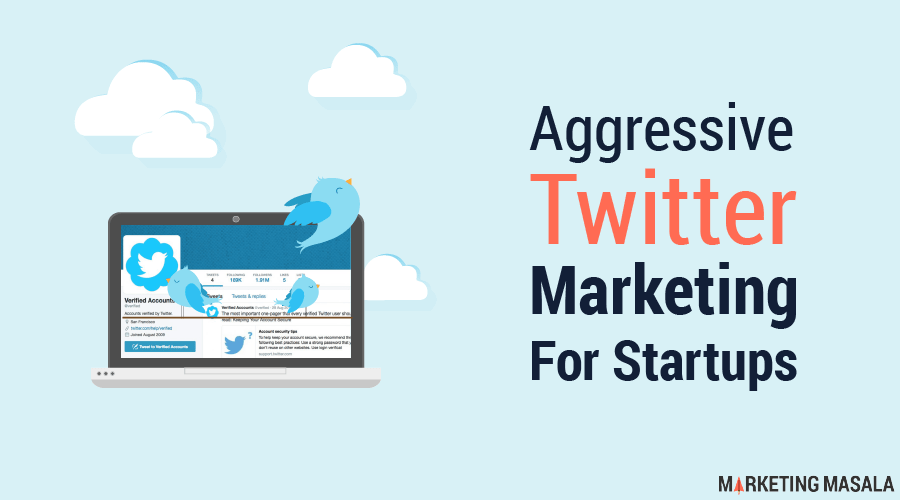The image features a rectangular shape filled with a light pastel sea breeze color, a delicate blend of green and blue hues. On the left side, there are four clouds—two smaller clouds in the front and two larger ones in the back, with one cloud higher than the others on the right side.

Prominently displayed in the center is a laptop with a gray base and a dark gray outline around the screen. The laptop screen itself has a teal background, adorned with multiple Twitter bird logos in various spots, indicating a social media theme. 

To the right of the image, text appears in different colors and fonts, starting with the word "Aggressive" in black with a capital 'A.' Beneath that, the word "Twitter" is written in orange with a capital 'T.' Following that, the word "Marketing" is in black with a capital 'M.' Directly below, "for" is written in capital letters "F-O-R" in black, and lastly, the word "Startups" is capitalized with an 'S.'

At the bottom of the image, the text "Marketing Masala" is displayed, with "Masala" spelled out as M-A-S-A-L-A.